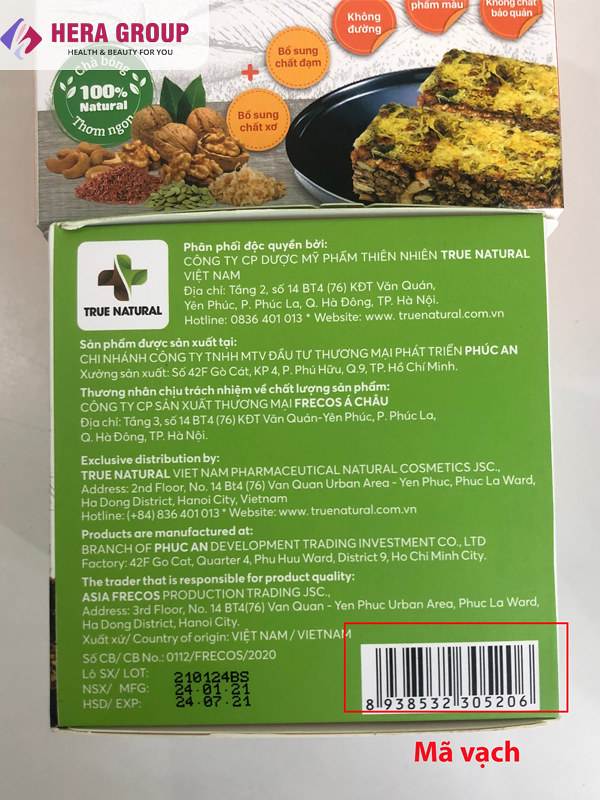This image showcases the back of a food package with a light gray background. The package itself has a green body with a white top and prominently displays the company's name, "Hera Group," in red lettering at the top left corner, accompanied by the tagline "Health and Beauty for You" in green. Below this, there is a green circle with white letters stating "100% natural." Just beneath the circle, there are various grains and seeds visible in orange, brown, and green hues.

To the right side of the package, there is a depiction of a black pan containing two squares of a yellow and brown layered food item, resembling lasagna or a similar dish with the top possibly being melted cheese. Below this image, on the green background, white text in various languages details the address for this Vietnamese product.

At the bottom of the package, a barcode is encircled in red, with the text "MA V ACH" in white with black lettering next to it. The expiration date printed on the package is "24-07-21." Additionally, the packaging includes information on natural cosmetics and distribution addresses, emphasizing the brand's message of being "True Natural."